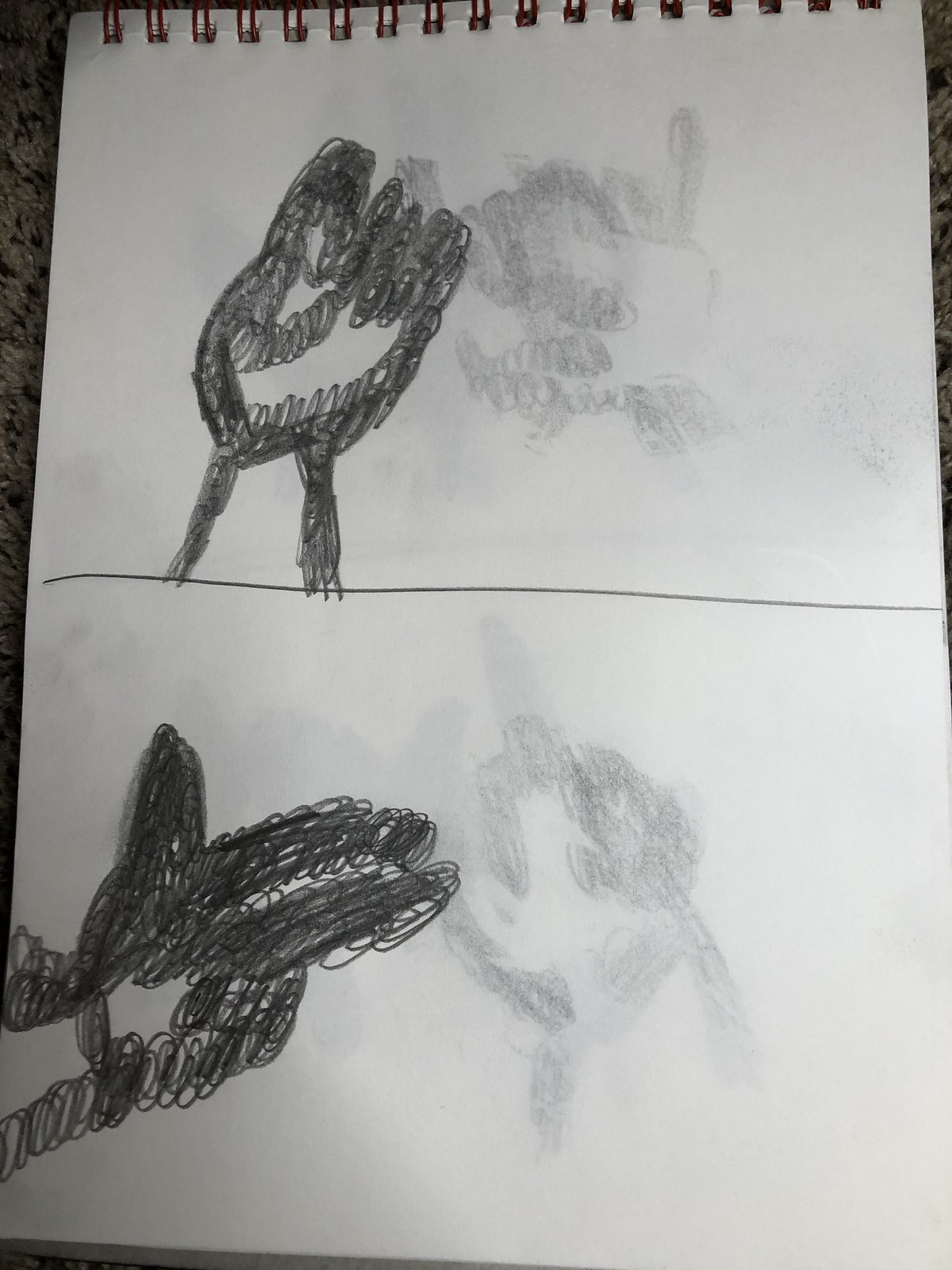A detailed photograph captures a meticulously sketched drawing within a spiral-bound notebook, prominently displayed against a subtle background of dark gray granite at the edges. The notebook's top spiral is visible, indicating its position in the frame. The paper is divided horizontally by a distinct dark pencil line, creating a top half and a bottom half for the illustrations. In the upper section, a dark pencil sketch depicts a hand with fingers closed towards the palm, facing directly towards the viewer, complete with a shadow cast on the back. In the lower section, an equally detailed sketch portrays the same hand, but this time positioned with the index finger extended and thumb raised, resembling a finger gun gesture. The intricate loops and shading techniques give a sense of depth and realism to both sketches.